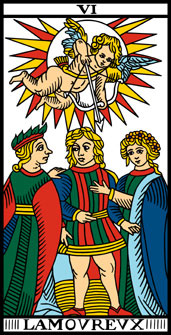This vividly colored painting, reminiscent of a tapestry, features a celestial scene. At the top, an angelic figure resembling Cupid is suspended mid-air, his bow drawn with an arrow aimed downward. Behind him, a radiant white sun with orange and yellow rays illuminates the scene. A banner above reads "VI," while the text at the bottom displays "L A M O V R E V X."

Below Cupid, three blonde-haired figures stand in regal attire. Central is a king, flanked by a lady on his right and a gentleman on his left. The gentleman on the left dons a red headband adorned with green leaves, complementing his green, red, blue, and yellow cape. The king is dressed in a similarly multicolored outfit, featuring hues of green, red, yellow, and blue. The lady on the right, distinguished by her distinct attire, wears a blue and dark blue cape over a similarly vibrant ensemble. The scene captures a moment of divine intervention or blessing by Cupid, poised above these dignified figures.